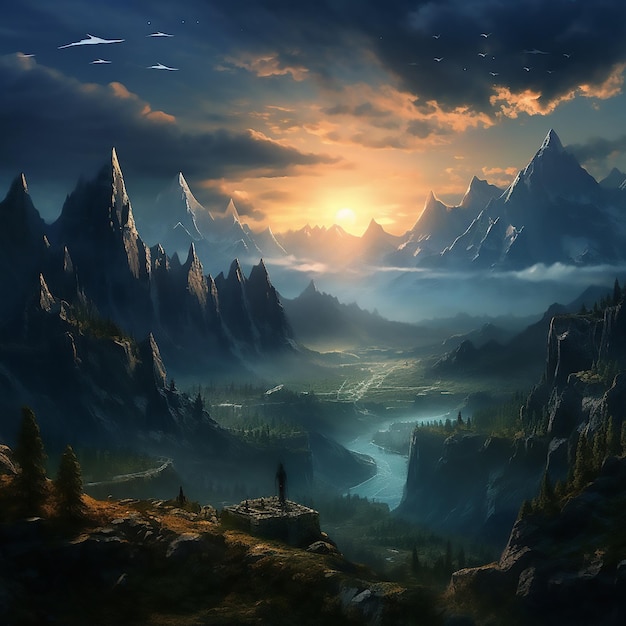The detailed image appears to be an artist's digital rendition of a fantastical world, possibly for a video game or a poster. Dominating the scene, a man stands on a square platform or structure atop a hill, gazing out over a landscape that features multiple, exceptionally steep mountains with sharp curves stretching into the distance. A dark blue sky hosts a dramatic sunrise or sunset, with the sun glowing white and yellow, radiating orange hues across the horizon. A mist envelops the entire landscape, creating an ethereal atmosphere. Green trees and shrubbery nestle beneath the mountains, with a wavy, light blue river cutting through a brown, rocky terrain in the center of the composition. The middle ground is clearer, revealing a detailed portrayal of nature intertwined with fantasy elements.